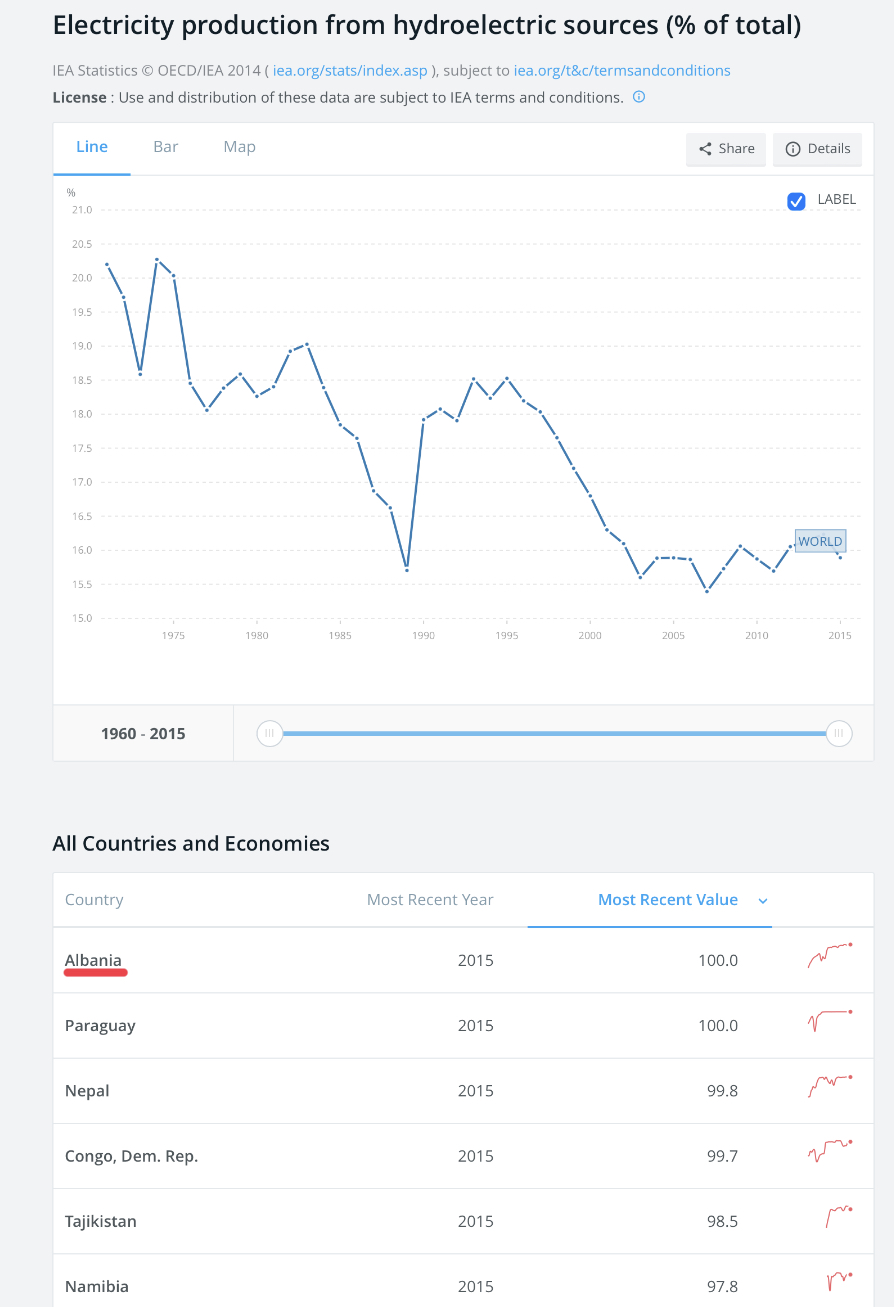This image features a detailed infographic titled "Electricity Production from Hydroelectric Sources (% of Total)" in bold black font, placed against an off-white background. Beneath the title, there is a small, hard-to-read black text followed by some turquoise text indicating it is subject to a license. It then states, in bold black font, the word "License" and in black font that the use and distribution of the data are subject to IEA terms and conditions, denoted by a small turquoise circle.

The first main section of the infographic is a vertical rectangular graph with a crisp white background. At the top of this section, there is a label "Line" in turquoise with an underbar, alongside "Bar" and "Map" which are grayed out. Right-hand icons accompany the header. The graph itself, depicted in blue, displays fluctuating data from 1960 to 2015, though the specific details are unclear. The x-axis shows a timeline from 1960-2015, corresponding to the off-white section, and a turquoise line runs horizontally from this axis.

The subsequent section, titled "All Countries and Economies" in bold black font against the off-white background, lists data in a table format with headings: "Country," "Most Recent Year," and "Most Recent Value" (highlighted in turquoise and underlined). 

Under the "Country" column, the countries listed include:

1. Albania
   - Year: 2015
   - Value: 100.0
   - Features a thick red underline and a small red line graph beside the value.
   
2. Paraguay
   - Year: 2015
   - Value: 100.0
   
3. Nepal
   - Year: 2015
   - Value: 99.8
   
4. Congo, Dem. Rep.
   - Year: 2015
   - Value: 99.7
   
5. Tajikistan
   - Year: 2015
   - Value: 28.5
   
6. Namibia
   - Year: 2015
   - Value: 97.8

The countries, years, and values are presented consistently in black font.